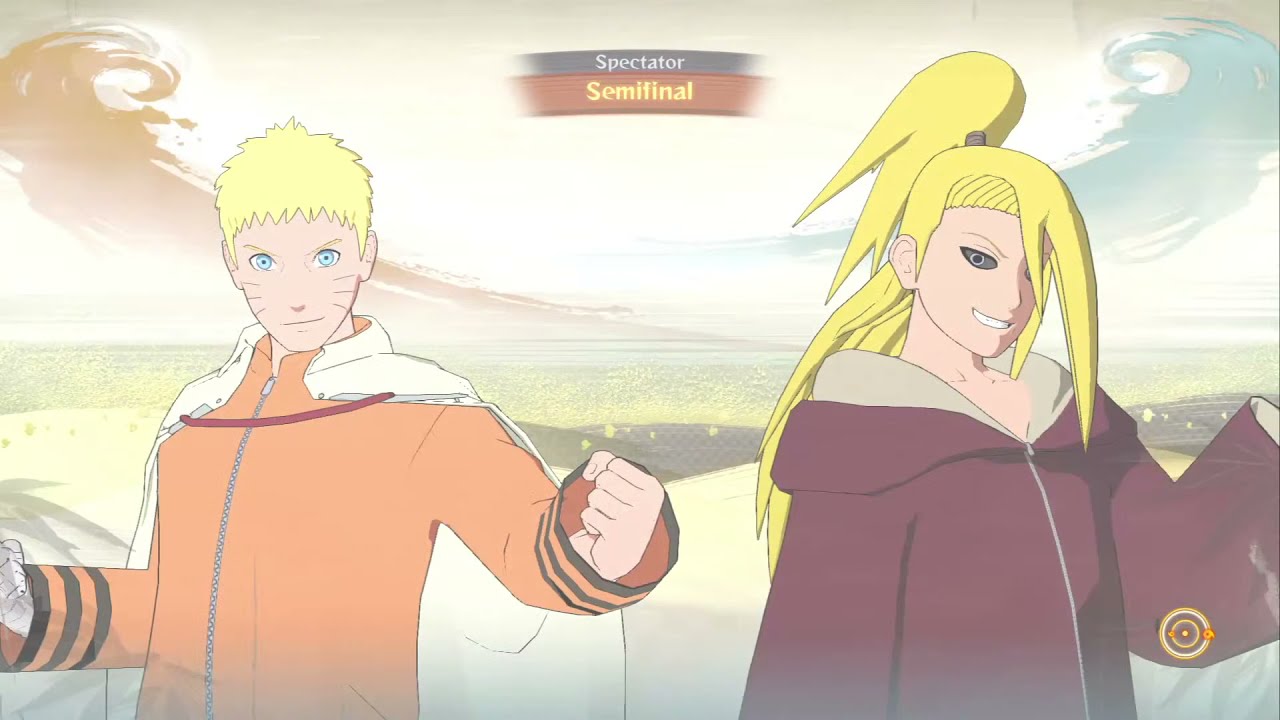The image is a detailed color illustration in an anime style, showcasing two characters set against a picturesque background. On the left stands a fair-skinned male with short, bright yellow hair, blue eyes, and distinctive cat-like whisker marks on his face. He wears an orange zip-up top with long sleeves, marked by three black rings around the cuffs, and is draped in a white cape fastened with a red cord. His pose is aggressive, with both fists raised in the air.

On the right is a female character, also fair-skinned, with long, bright yellow hair styled in a high ponytail that cascades down her back and partially covers her face. She has dark eyes and wears a maroon zip-up top with large sleeves and a hood lined in beige, resting on her back. She stands smiling, with her left hand raised.

The serene background features cartoonish structures, possibly stones, leading to an expansive meadow under a tall sky filled with swirling clouds. An in-image banner between the characters reads "Spectator Semi-Final," hinting at an impending battle or competition.